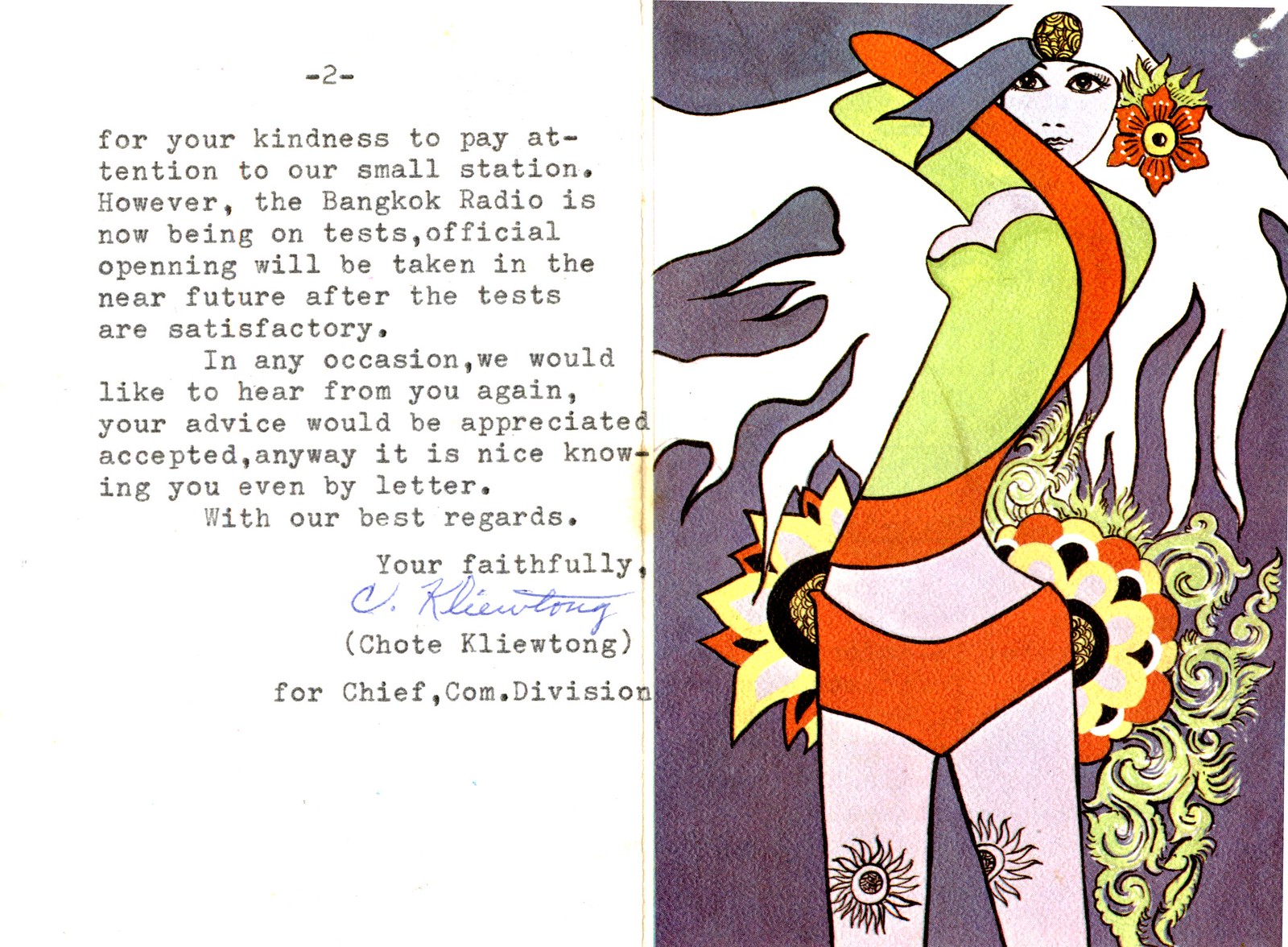This detailed poster is split vertically into two parts. The left side features a typewritten letter marked as page two. The letter begins with "For your kindness to pay attention to our small station," and mentions that "Bangkok radio is now being on test." It proceeds to state that the official opening will follow once tests are satisfactory, and expresses a desire to hear from the recipient again. Closing with "With our best regards, yours faithfully," the letter is signed by Chote Klutong, identified as being "for Chief, Comm Division."

The right side displays a vivid watercolor-style portrait of a woman against a predominantly purple background. She has long, flowing white hair adorned with a large orange flower near her ear on the left side. Her forehead features a circular gem, and she has dark, striking eyes and eyebrows. She wears a green top that transitions into an abstract swirled yellow pattern covering her upper torso, paired with orange bikini bottoms. Her legs, visible to the knees, are decorated with circular, sunburst-like tattoos. Additional design elements resembling flowery petals emanate around her legs, adding to the imaginative and colorful composition. Overall, this section of the poster is rich in orange, purple, black, and yellow hues.